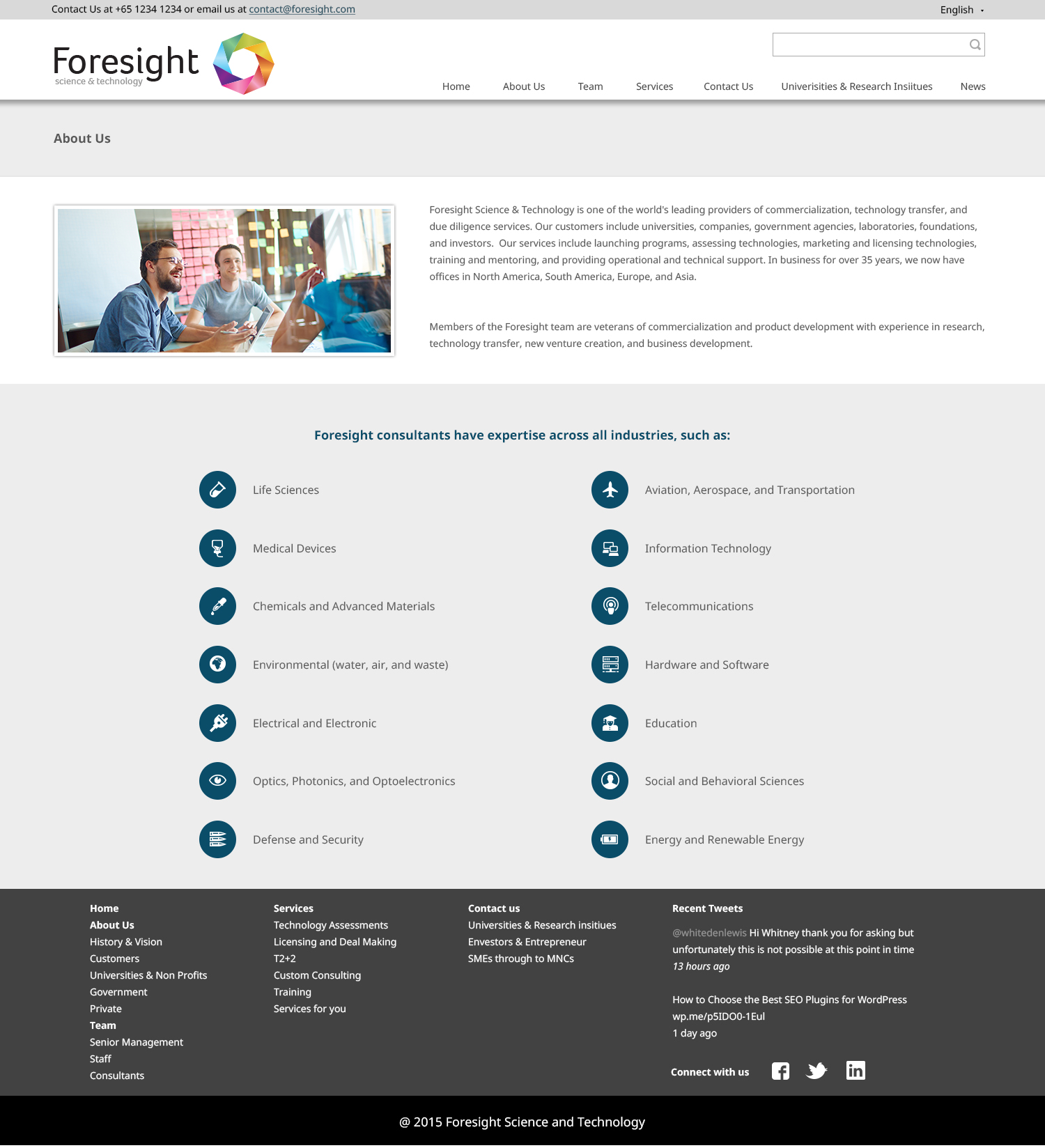Screen capture of the Foresight website showcasing its header with contact information, including an 800-number and an email address. Prominently displayed is an octagon ring with multiple colors, symbolizing diverse expertise. The website's "About Us" section features an image of casually dressed individuals in t-shirts seated around a conference table, engaged in discussion. Accompanying text highlights Foresight Science and Technology as a leading provider in several fields. Detailed descriptions mention expertise in life sciences, medical devices, defense and security, aviation, aerospace, transportation, information technology, telecommunications, hardware, software, and more, illustrating the broad industry reach and capabilities of Foresight Consultants.